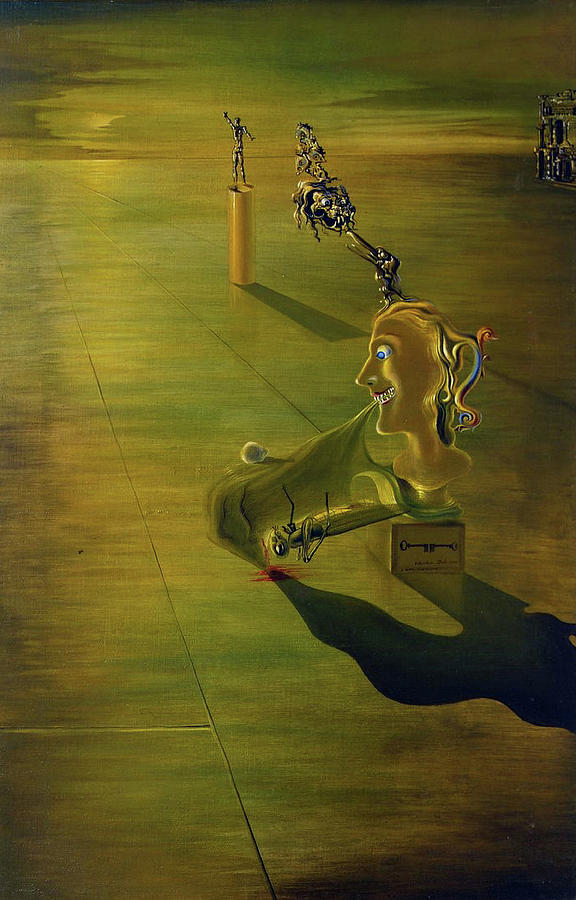This macabre and unsettling painting evokes a sense of eerie surrealism, reminiscent of Salvador Dali's work. The scene is set against a gloomy green background, with dark, foreboding skies that heighten the painting’s creepy atmosphere. Dominating the composition on the right side is a man's head, positioned like a bust on a small stand atop a wooden box adorned with two keys facing one another. The head features a curious detail – a cloth clutched between its teeth, ending in what appears to be a skull. 

In front of the head, a grasshopper or possibly a cricket lies on its back, enveloped by smoke or fluid emanating from the mouth. Both surreal and cryptic elements add to the painting's mystery. In the background, a line of flying insects approaches ominously, while strange shapes populate the surreal landscape. There seems to be a humanoid figure standing on a tall cylindrical pedestal, and not far from it, a hybrid monstrous dog advances towards a bird. Additionally, the distant right side features what looks like the facade of a temple, adding to the enigmatic, infinite terrain that resembles poured concrete or stone slabs. The overall color palette is a haunting blend of greenish, yellow, and brown hues, completing the eerie and thought-provoking tableau.